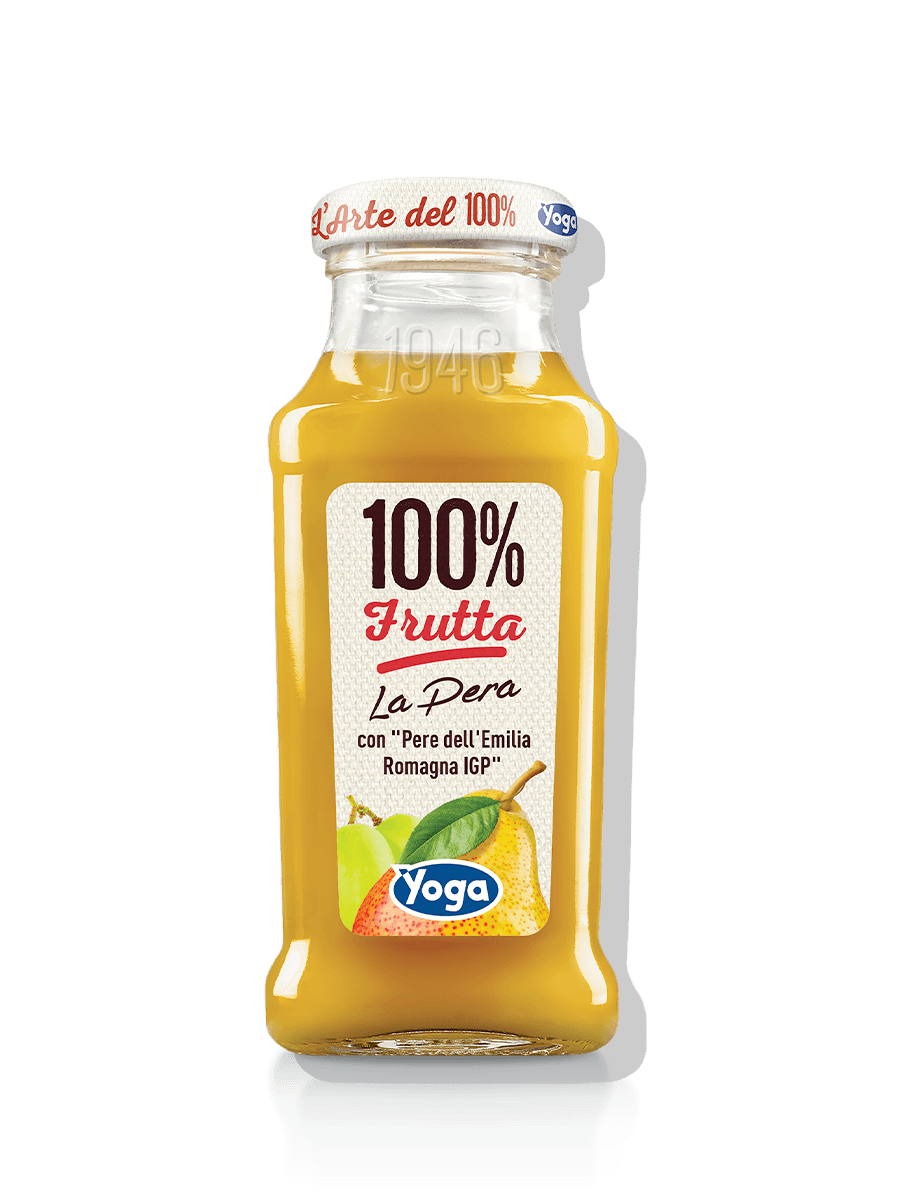The image showcases a rectangular, square-shaped glass bottle, centrally positioned against a white backdrop, casting a slight shadow. The bottle features a white twist-on metal cap adorned with red text that reads "La Arte Del 100%," accompanied by a blue oval logo with the white text "Yogo." The neck of the bottle bears the semi-transparent number "1946," giving it a vintage touch. The bottle contains an orangish-yellowish substance, suggestive of fruit juice or a smoothie.

The front of the bottle displays a gray label with multiple lines of text. At the top, black text reads "100%," followed by red cursive text with a red underline stating "Fruita," referring to fruit. Just below, smaller black text reads "La Pera," which translates to "the pear." Further down, in even smaller text, it says "Con Pera Della Emilia Romagna IGP," indicating the use of pears from the Emilia Romagna region of Italy, known for specific quality-controlled products.

The label also features an illustration of a large yellow pear with a green leaf and brown stem. Off to the left, the label depicts two green pears connected by a single stem. All these elements come together to present a product that emphasizes its 100% fruit content and regional authenticity.